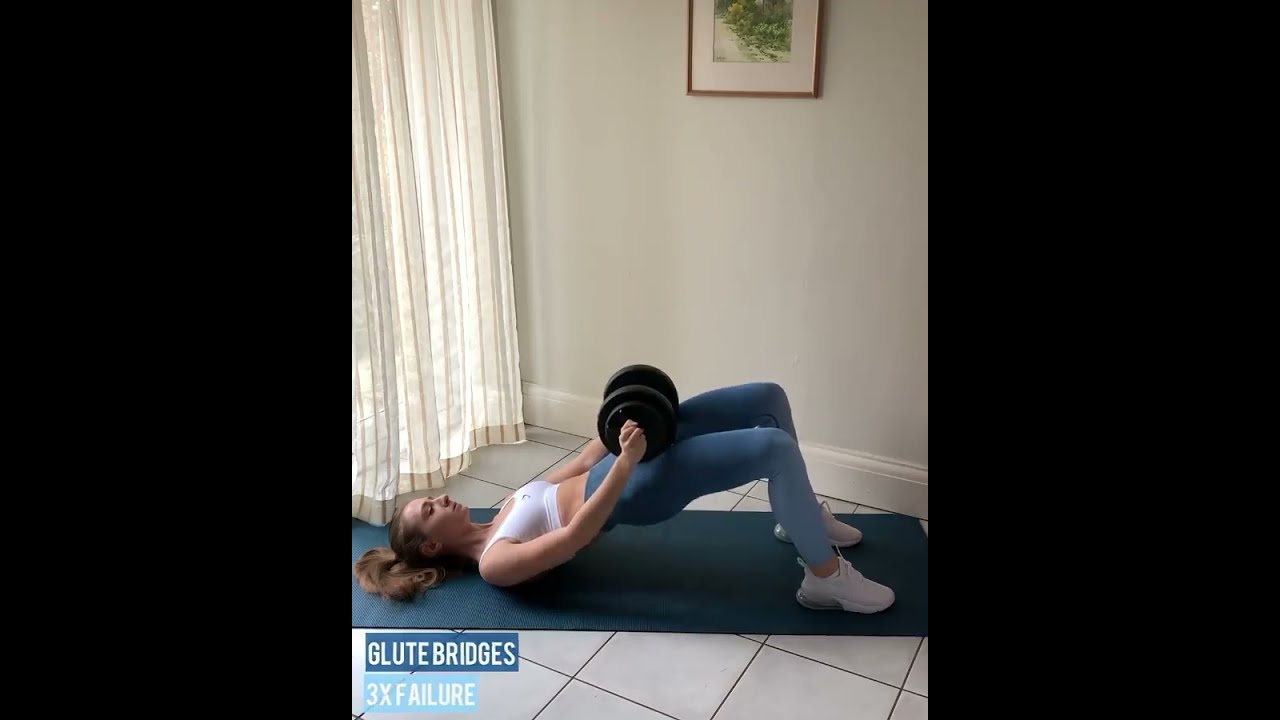In the image, a fit and muscular woman is performing an exercise known as a glute bridge on a blue exercise mat laid out on white tile flooring. She is dressed in a white sports bra and blue stretchy spandex pants that are darker at the top and lighter at the bottom, paired with white sneakers. The woman has her shoulders and feet planted firmly on the mat, with her knees bent and hips thrust upwards. She holds a heavy black dumbbell with both hands positioned over her hips. Her head, adorned with a ponytail, rests on the mat, and the entire scene appears to be set in a home environment with white walls and large white tiles. Behind her is a white curtain featuring light brown vertical stripes, and a picture frame on the wall displays greenery with a brown border. The lower left corner of the image contains a caption that reads "GLUTE BRIDGES 3X FAILURE" in white font against a blue background, with "GLUTE BRIDGES" on a darker blue section and "3X FAILURE" on a lighter blue section.